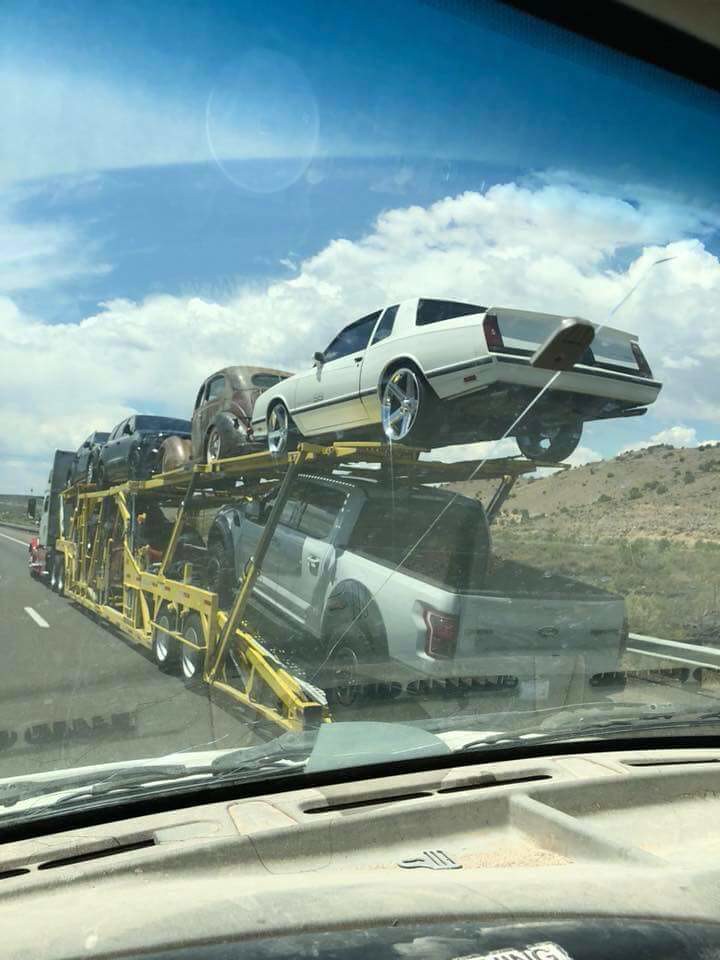This photo, taken from inside a high-sitting vehicle such as an RV or truck, captures the view through a cracked windshield revealing the dashboard and windshield wipers. The scene outside shows a double-deck vehicle transporter truck painted in yellow, carrying several cars on a highway. On the bottom level at the back, there is a gray double-cab pickup truck, possibly a Toyota, and multiple indistinguishable vehicles in front of it. The top level showcases a white 1970s style car with large, oversized rims, and a very old-fashioned 1930s car with a domed cab and protruding wheel wells, reminiscent of a classic gangster vehicle complete with running boards. In the distance, the white and red cab of the transporter truck can be seen. The highway is flanked by grassy plains and hills on the right, with a typical American corrugated steel guardrail. The blue sky is dotted with large, anvil-bottom cumulus clouds, adding to the clarity of this bright, sunny day.